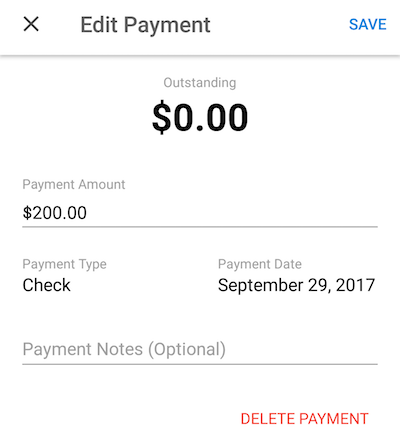The image is a detailed screenshot of a payment interface from a website or app. At the top, there is a row of icons including an 'X' to cancel, an edit option, and a 'SAVE' button in blue. Below these options is a thin gray line spanning the width of the screen.

Following this, the section labeled "Outstanding Balance" is presented, with "Outstanding" in gray and an amount displayed as "$0.00 USD." Moving down, the "Payment Amount" section is highlighted, with its title in gray and set with initial capital letters. This section allows users to enter a payment amount, shown here as "$200."

Another thin gray horizontal line separates the sections. Next is the "Payment Type" category, also in gray with capital letters for the initial words. Underneath it lists "Check" as the chosen payment method.

Below is the "Payment Date" category in gray, indicating the date as "September 29th, 2017." Following this section is "Payment Notices" in gray, with "optional" indicated in parentheses.

The last element is a thin gray line underlining the previous sections, leading to the "DELETE PAYMENT" option at the bottom right corner of the interface, highlighted in red capital letters.